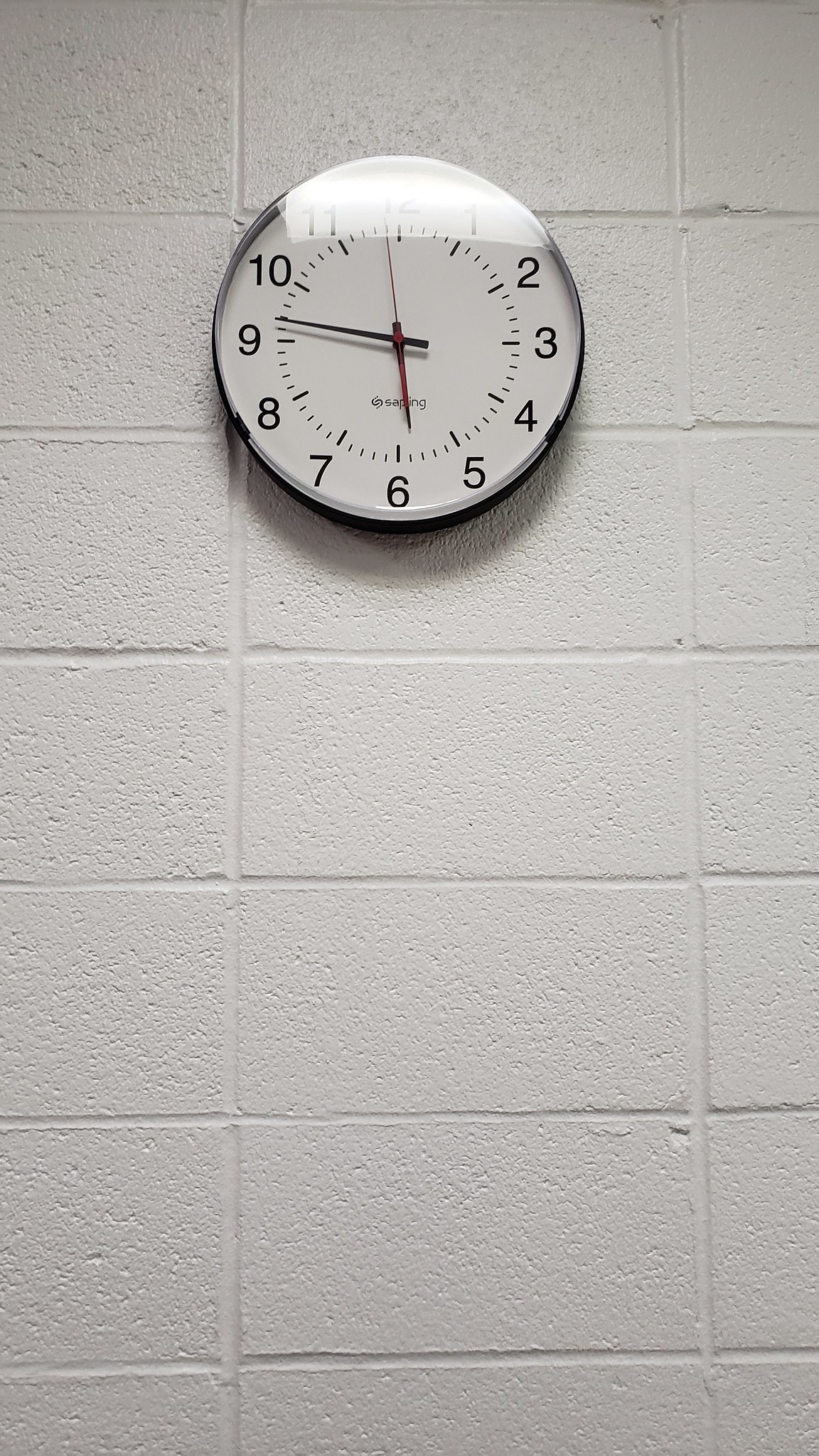This photograph captures a circular wall clock mounted on a white-painted cinder block wall. Positioned centrally in the upper portion of the image, the clock features a clean, white face accented by a thin black border around its circumference. The black numbers, arranged around the outer edge of the clock face, provide clear indicators of the hours. Inside the numerical ring, minute and hour markers are represented by thin black lines, with the hour markers appearing longer and bolder for easy distinction. The clock's hands, also in black, contrast sharply against the white backdrop, while the second hand stands out in a vivid red. A subtle reflection of light at the top of the clock partially obscures the number 11, while the numbers 12 and a portion of 1 remain visible, adding a touch of realism to the image.